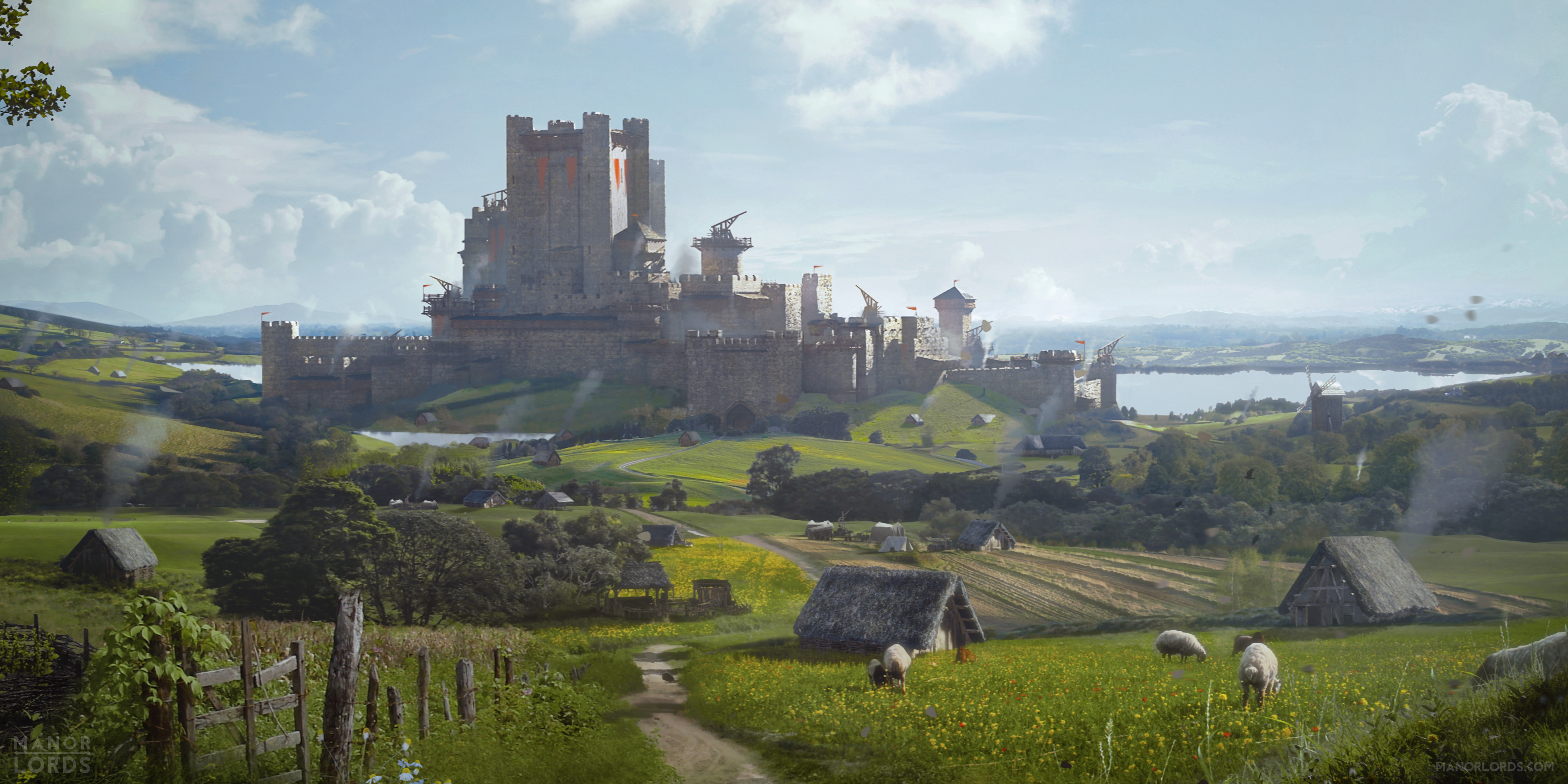The image depicts a sunlit, expansive landscape centered around a large, medieval castle that dominates a walled partial city. The castle, squarish and imposing with multiple towers, appears somewhat aged, with parts seemingly worn down over time. Surrounding this towering structure are numerous smaller dwellings, ranging from simple triangular-roofed homes to basic cabins, each constructed with a thatched roof that hints at a medieval setting.

Lush, vibrant green grass extends across the landscape, dotted with patches of agriculture and grazing sheep. Fragmented wooden fences, some falling apart, are scattered near the foreground, adding to the rustic charm. The bottom left corner bears the printed words "manor boards." Beyond the castle and its surrounding homes lies a large, glistening lake under a light blue sky with a few white clouds. The entire scene, possibly a detailed drawing rather than a photograph, exudes a sense of historical serenity and timelessness.